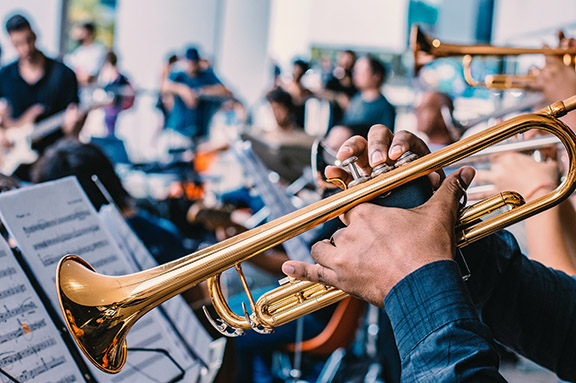In this image, you see a close-up of a person playing a brass-colored trumpet, their hands clearly visible and adorned in a long-sleeved blue shirt. The focus is on the player, whose upper body and head are not visible. Positioned in front of the trumpet player is an open book of sheet music, resting on a music stand.

The background reveals a busy interior environment, indicative of a band practice session or orchestral rehearsal. Blurred but discernible, various musicians are engaged with their instruments. To the left, a man is playing guitar, while additional trumpeters are scattered throughout the scene. The backdrop features what appears to be white walls or screens, adding to the indistinct bustle of the setting. Various music stands with scattered sheets of music contribute to the active and lively atmosphere.